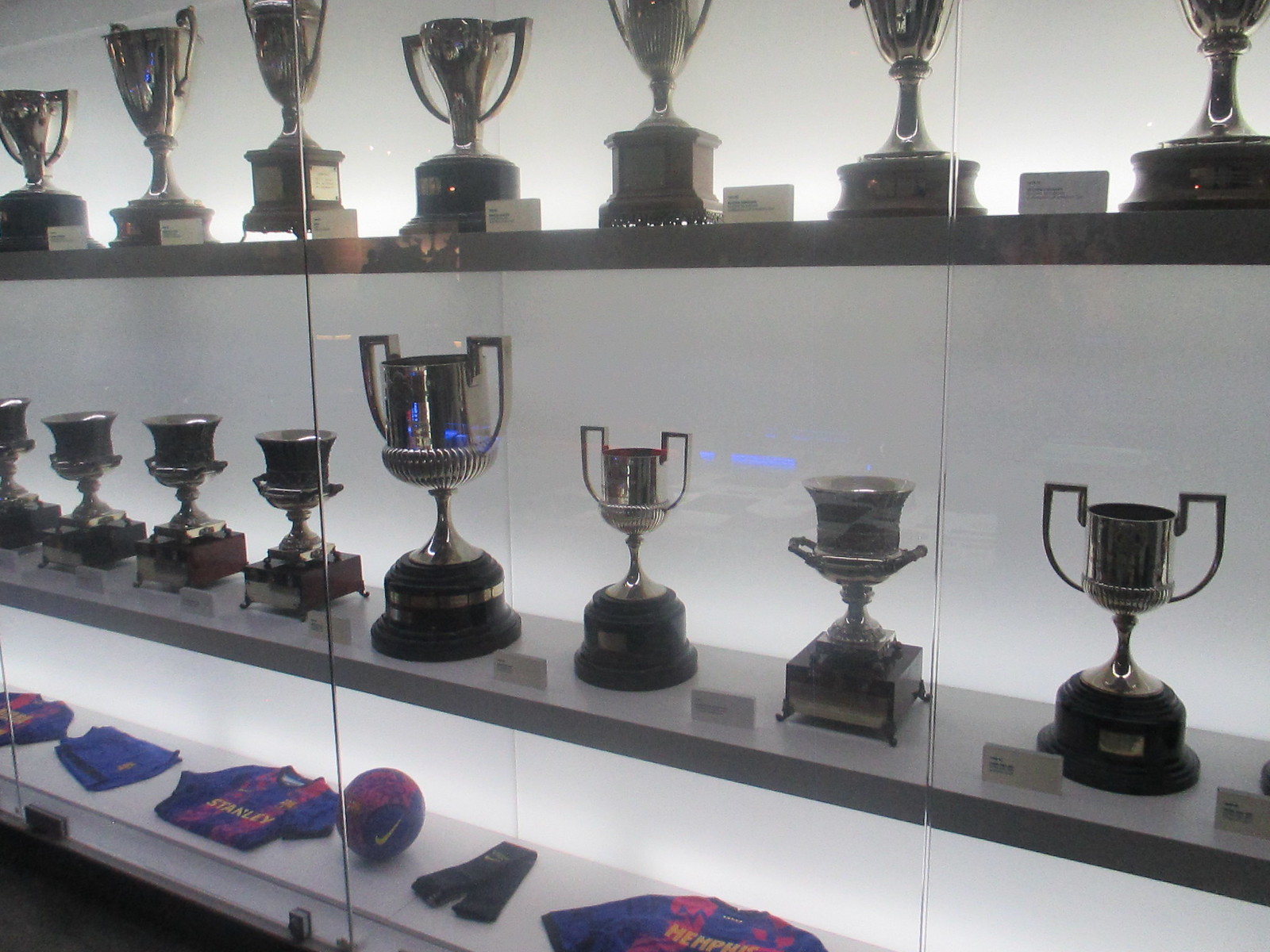The image displays a well-organized trophy case with three shelves, viewed through a glass front. The case is backlit with a white light, enhancing the shine of the items inside. The top shelf is lined with an array of silver trophies, each with handles, and unique shapes and base styles, some round and some square. The middle shelf also holds an assortment of shiny metal trophies, smaller in size with prominent wooden bases, arranged uniformly with small white cards placed slightly to their left. The bottom shelf features various sports paraphernalia including a blue uniform with red stripes and the name "Stanley," a multicolored soccer ball adorned with a Nike checkmark, folded soccer jerseys, gloves, socks, and shorts. The base of this shelf is white, contrasting with the dark wood of the upper shelves. The case is secured with a visible lock on the front glass door.